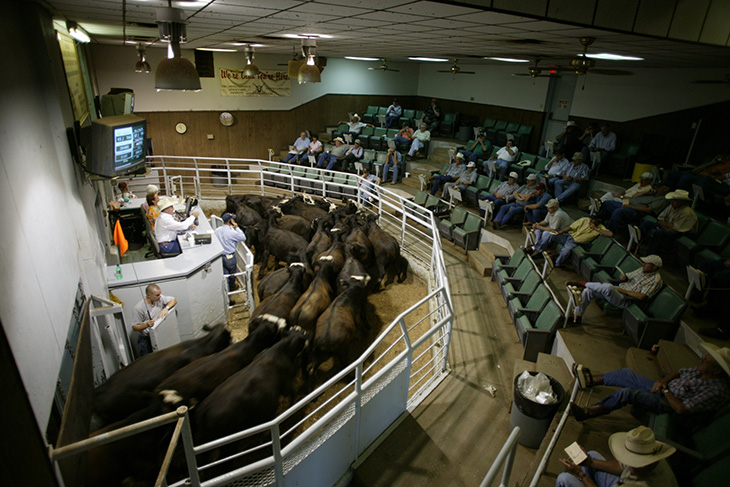This photograph captures a bustling cattle auction set in an arena with white walls and wood paneling extending halfway up. From the top left corner, we look downward to the right. Approximately 50 green theater-style seats form a half circle on the right, with about 30 people, mostly men in cowboy hats, rancher hats, or baseball caps, and dressed in jeans and casual shirts, occupying them. The central focus is the white-fenced cattle pen on the left, where dark brown and black cattle are moving from the bottom left upward in a circle. Behind the cattle, a cowboy in a white shirt and jeans, wearing a cowboy hat, is seated. Above him is a television screen. The environment is lit by overhead fluorescent lights, with a large trash can visible in the lower right corner of the image. The arena floor is a dark ecru tan color, enhancing the rustic feel of this vibrant auction scene.